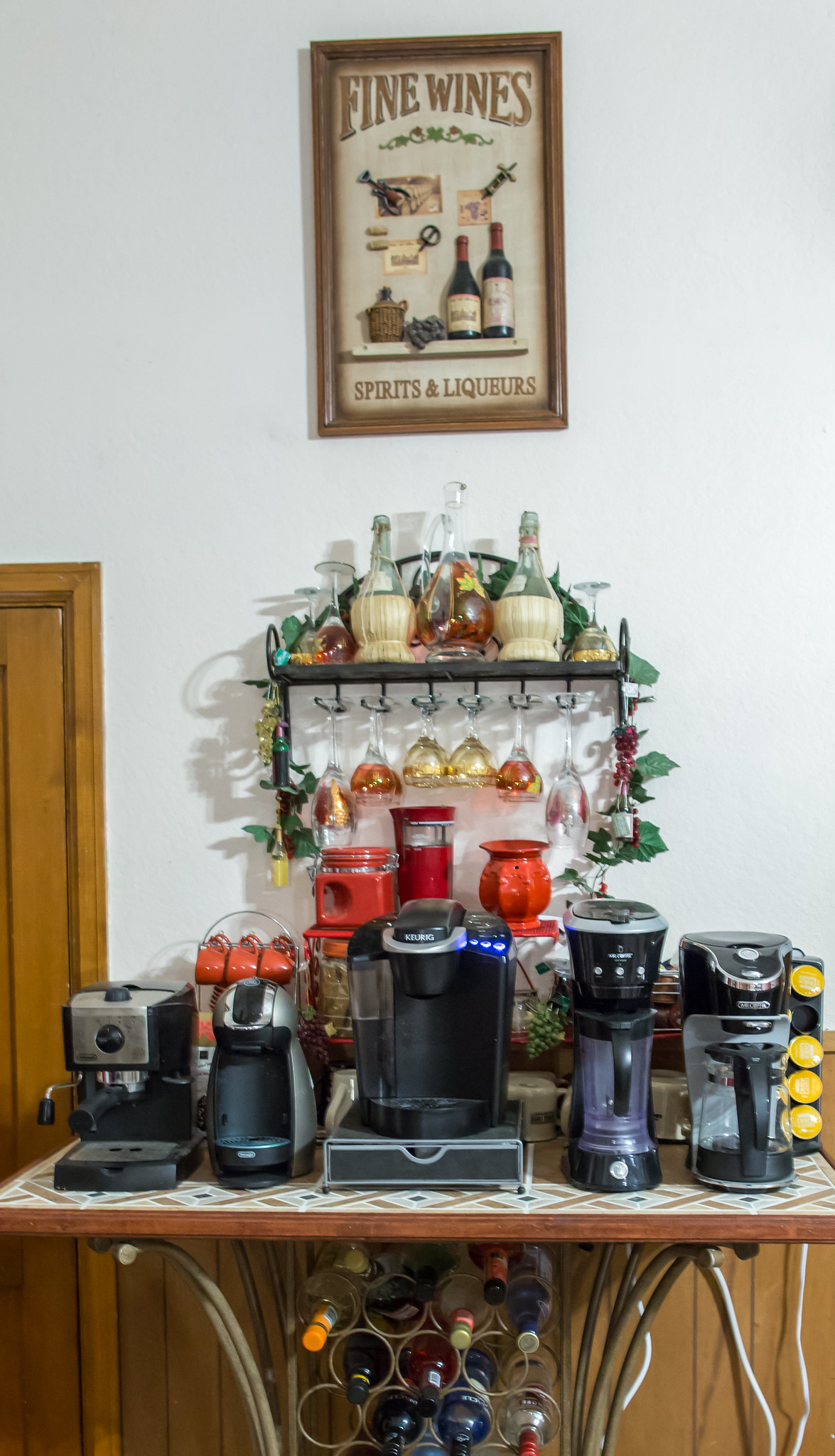The photograph depicts a detailed setup within a room showcasing an organized wine and coffee station against a white wall. Central to the image is a table with wooden trim and an inlaid tile top, featuring a variety of beverage-related items. Beneath the table, there is a wine rack filled with numerous bottles of wine, supported by gold metal legs. On top of the table, five different coffee makers are displayed: two unbranded on the left, a Keurig machine in the middle, and two Mr. Coffee machines to the right of it. 

In the background, a collection of white coffee cups is neatly lined up, along with a red coffee grinder, and various red containers. A small silver rack holds more red coffee mugs, and a black stand is filled with coffee pods for the Keurig machine. Adding to the ambiance, a metal rack is mounted above the table; it features a top shelf holding several wine bottles and upside-down wine glasses, with small glass fruits hanging from it as decoration.

Above this setup, a framed sign reads "Fine Wines, Spirits, and Liqueurs" against a beige background with a wooden frame. The sign is adorned with illustrations of grapes and wine bottles, contributing to the old-timey feel of the space. This area is meticulously arranged to serve as both a coffee and wine station, blending functionality with aesthetic appeal.